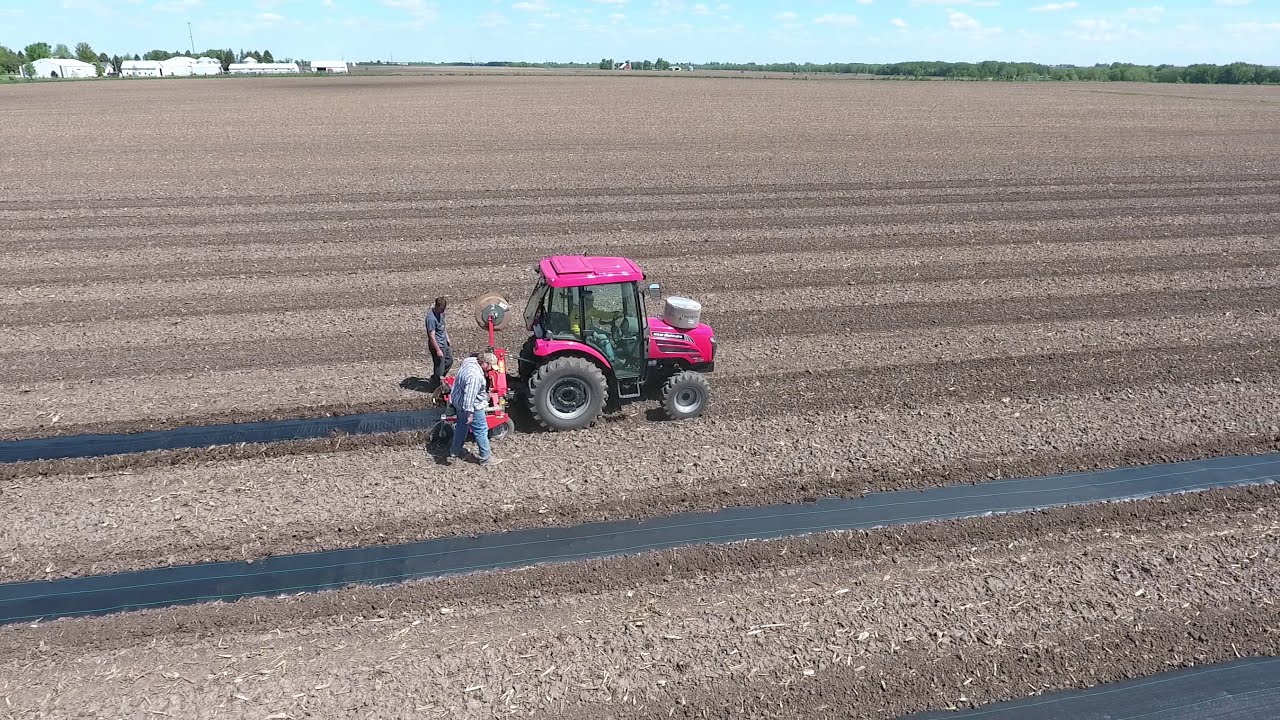In the rectangular photograph of a vast farmland, the foreground depicts a recently tilled field with distinct, darker tilled rows running horizontally across the soil. At the center of the image is a pink tractor, characterized by its pink roof, fenders, and front engine cover. The tractor's rear tires are notably larger than those in the front, and its cab features a transparent opening through which a person in a yellow shirt and blue pants can be seen driving. Two individuals walk behind the tractor; one wears a white shirt with stripes and blue jeans, while the other dons a dark gray shirt and dark pants. The tractor appears to be laying down strips of black plastic, as seen where the rows alternate between bare soil and plastic-covered strips. In the far distance, the upper left corner reveals tiny, white barn-like structures surrounded by bright green trees. Meanwhile, the right side of the background shows the edge of the field bordered by a tree line. The sky overhead is a light blue with scattered white and gray clouds, completing the serene, agricultural scene.